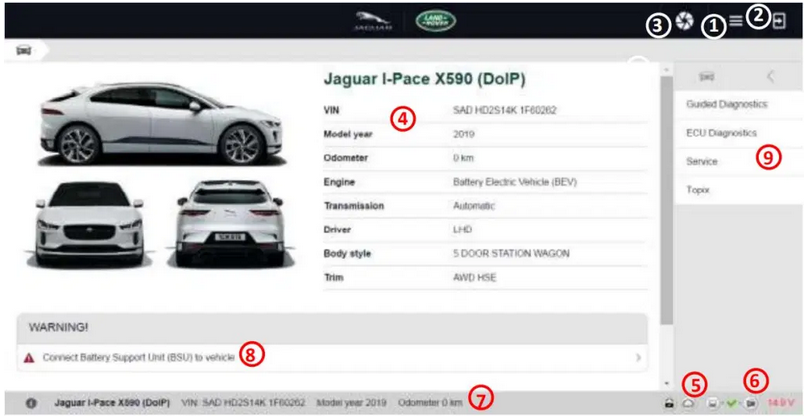On the car dealership website, a sleek and professional black banner tops the page, featuring prominent brand insignias and information. The left side of the banner displays the iconic Jaguar logo and name in bold text. Adjacent to this, the green, elliptical Land Rover logo is prominently displayed with "Land Rover" inscribed in white uppercase letters.

On the right side of the banner, a sequence of circular icons numbered 1, 2, and 3 is visible, suggesting some navigation or highlighting feature.

Below the banner, a high-quality image of a white Jaguar sedan with four doors is showcased. The sedan boasts a sleek back design, a compact front grille, and stylish silver alloy wheels, epitomizing elegance and modern automotive design. The page includes three photographs of the vehicle: a captivating side view, a striking front angle, and a detailed rear perspective that highlights the taillights and the signature Jaguar emblem.

To the right of these images, the vehicle's details are clearly listed in green text: "Jaguar I-PACE X590 (D-O-L-P)." Additional specifications include the VIN number, model year (2019), and odometer reading (0), indicating that the car is a new, electric vehicle. The engine type is battery electric, paired with an automatic transmission. The driver configuration is noted as LHD (left-hand drive). The body style is classified as a five-door station wagon with an AWD (all-wheel drive) trim, offering versatility and performance.

This well-organized and detailed presentation provides potential buyers with comprehensive insights into the featured Jaguar I-PACE, combining aesthetic appeal with vital technical information.